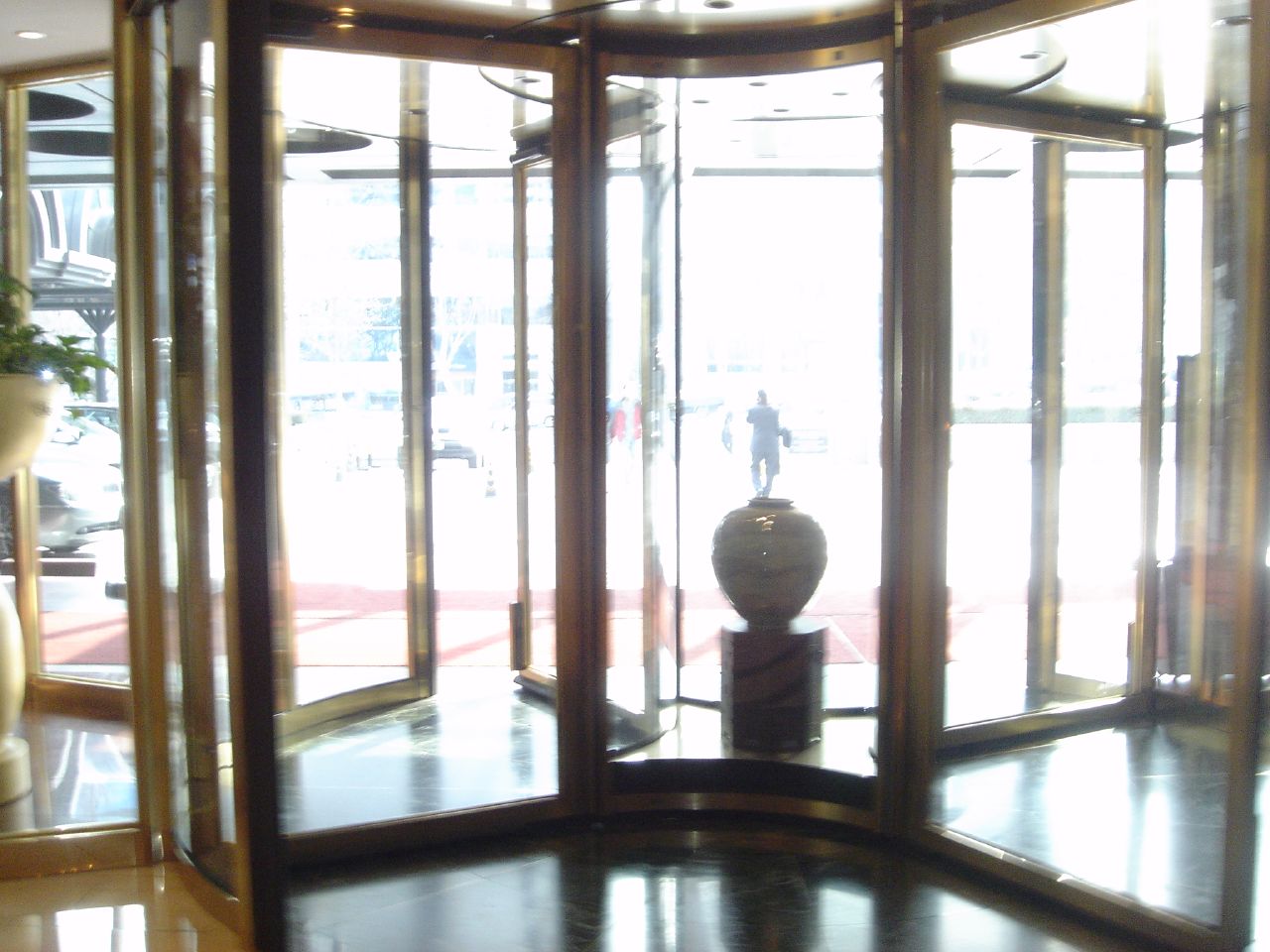The photograph captures an interior view of a large, ornate historical building, looking out onto a bright, sunny street. Dominating the composition is a set of revolving doors, their frames adorned with intricate brass or gold-like trim that exudes a sense of antiquated grandeur. Positioned centrally within the revolving doors is a statue, possibly a bust, standing atop a pedestal or vase-like structure. The ceiling above features recessed pot lighting that casts a subtle illumination, contrasting with the intense, almost blinding white light flooding in from outside. Through the glass doors, a few indistinct figures can be seen walking along the street, adding a touch of life to the vivid daylight scene. Additionally, a plant is located to the left side, contributing to the richness of the setting, which is likely a grand hotel or a similarly prestigious building.